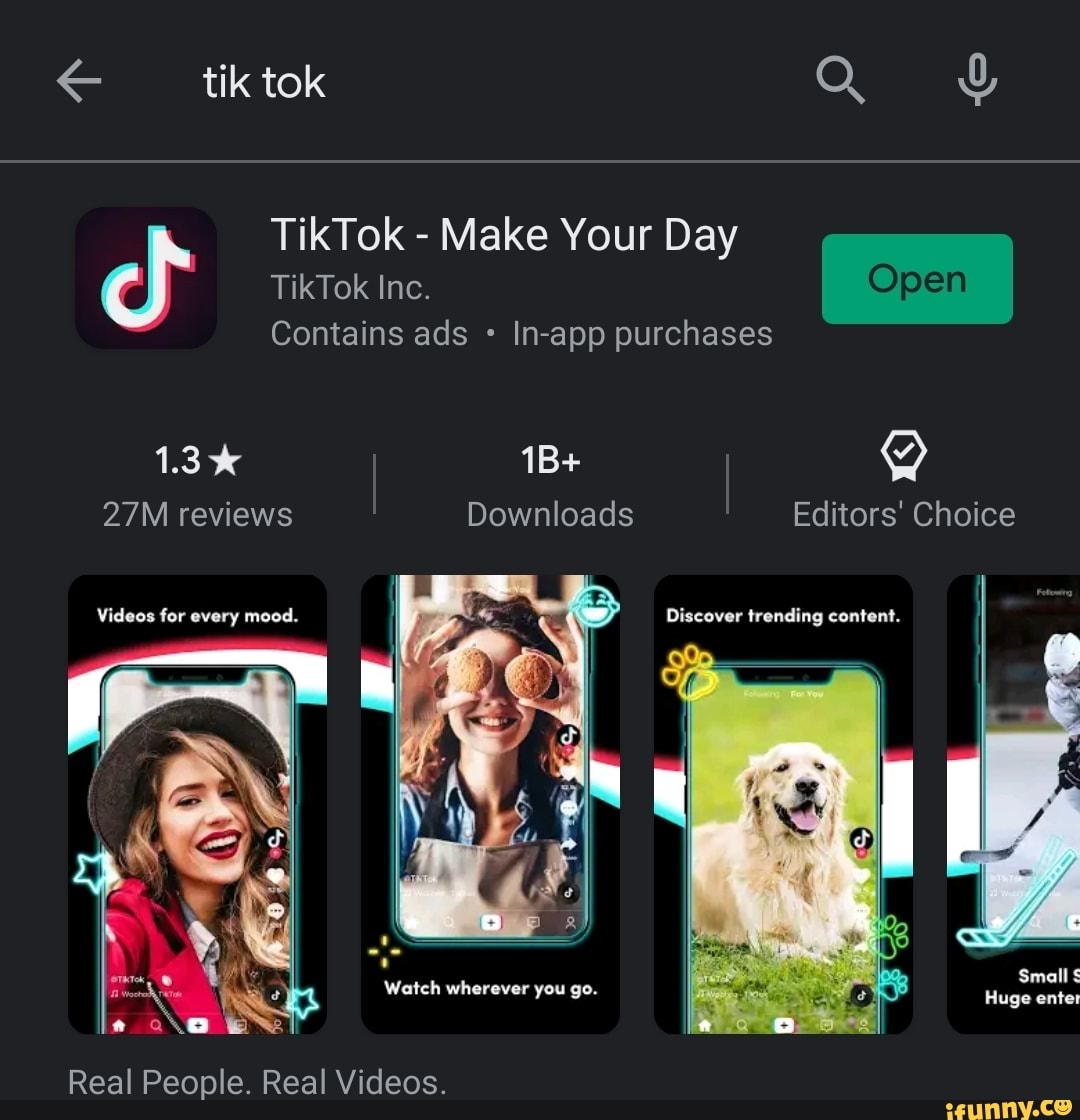**Detailed Caption for Advertisement Image:**

This advertisement exemplifies the mobile app "Tic-Tac," showcasing its interface and features. At the top of the promotional display, a user interface is illustrated where an individual has opted to search for "Tic-Tac." Alongside the search bar are icons including a left arrow for navigation, a search symbol, and a voice search option. Beneath this interface, prominently displayed, is the "Tic-Tac" logo accompanied by the tagline "Make your day." The app is indicated to contain ads and in-app purchases. Because the app has already been downloaded, the green button reads "Open;" otherwise, it would display "Download."

The app has received a rating of 1.3 stars out of 27 million reviews and boasts over 1 billion downloads. Notably, it is also marked as the “Editor’s Choice.” 

Below the general information section, the ad provides a preview of what users can experience with "Tic-Tac." The bottom left image features a stylish young woman in her mid-20s wearing a chic hat and a red jacket; the caption underneath reads, "Videos for every mood." Next to this is an image of a playful woman humorously using cookies as an eye mask, captioned, “Watch everywhere you go.” The subsequent image is labeled, "Discover trendy content," and depicts a panting dog in a field. The final preview image, partially cut off, shows an action shot of a sports activity involving hockey sticks and players chasing a puck. 

In the bottom right corner, a brand mark for ifunny.co is displayed in orange. Meanwhile, semi-discretely placed on the bottom left corner in white text on a black background is the slogan: "Real people. Real videos." This advertisement aims to convey a dynamic and entertaining user experience offered by "Tic-Tac."